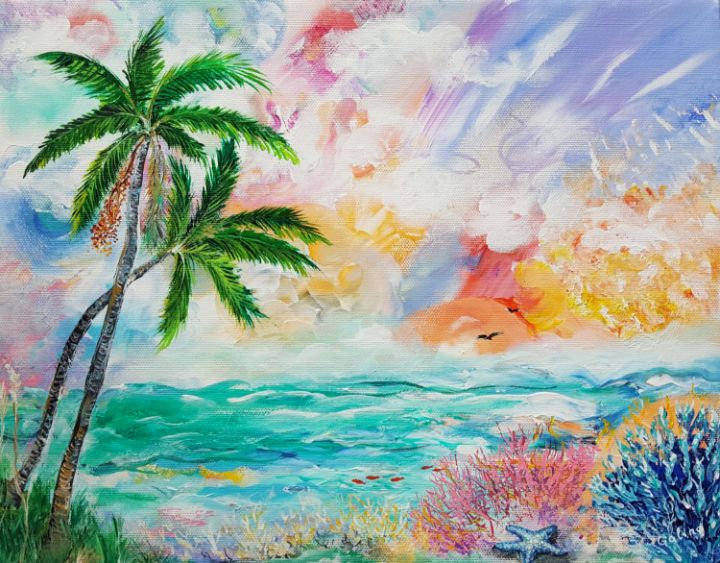This vibrant, colorful artwork appears to be a watercolor or oil painting depicting a tropical coastal scene. Dominating the left-hand side in the foreground are two tall, slender palm trees with brown trunks and bright green leaves. Surrounding the base of the trees is a carpet of green grass. Beside the trees, there is a stunning array of coral in hues of pink, blue, orange, yellow, and white, with a prominent blue starfish resting amongst them. Further to the right, small red fish can be seen swimming amidst the coral. The scene's midsection features dynamic, turquoise and blue waves, flecked with white to simulate foam, conveying the movement of water. Above the waves, the sky is an abstract swirl of colors, including blue, white, yellow, pink, purple, and bluish-green, blending seamlessly and creating a sense of wind and motion. Intriguingly, the sky even seems to reveal a faint impression of a human face, adding an element of mystery to the composition. The overall effect is one of lively, multicolored beauty, capturing the essence and vitality of an idyllic tropical seascape.